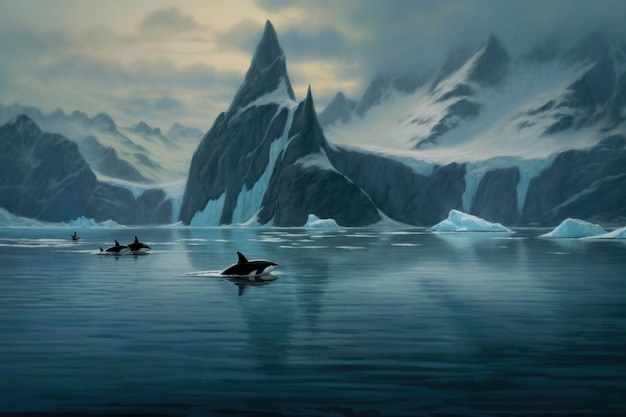This detailed painting depicts a fantasy-like ocean scene during a sunset or sunrise, characterized by a moody yet mesmerizing atmosphere. Three majestic killer whales are gracefully swimming from left to right in the frigid, blue water. The largest whale is prominently positioned in the center, with two slightly smaller companions trailing behind. They navigate a rugged, icy seascape dominated by a towering, pointed glacier in the middle. In the background, towering snow-covered mountains frame the scene, adding to the sense of grandeur. The sky above is a dramatic blend of heavy blue clouds tinged with hints of orange from the sun's elusive rays piercing through. The water and ice below shimmer with cold vitality, completing this intricate and evocative portrayal of nature's stark beauty.